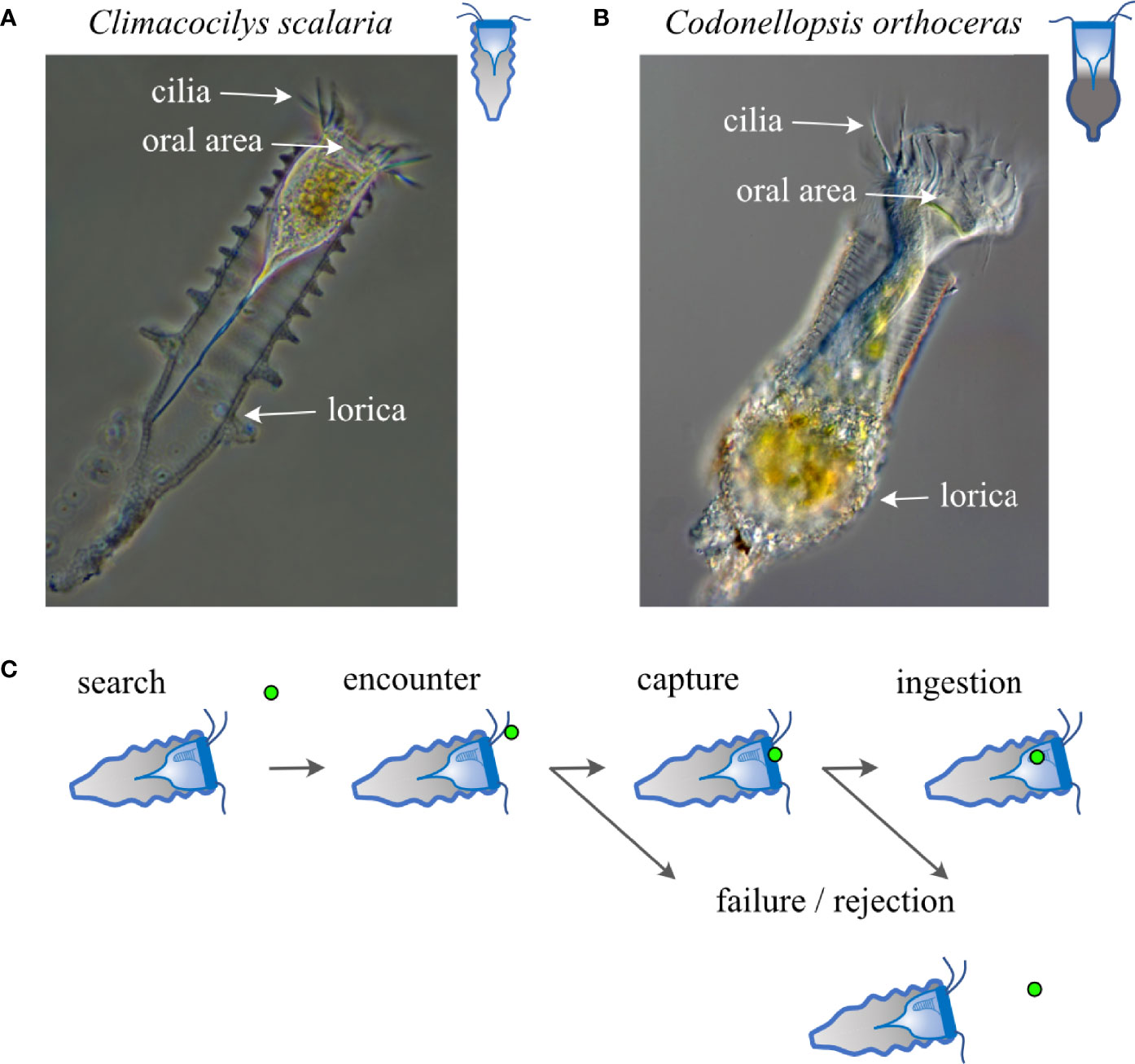The image consists of detailed photomicrographs and labeled diagrams of two microorganisms, *Climacocillus sclerum* and *Codonellopsis orthoceres*. In the left-hand photograph, *Climacocillus sclerum* is depicted with a cylindrical shape, tiny protrusions along its sides, tapering to a point at one end, and an opening with hair-like cilia at the other. Labels indicate its cilia, oral area, and lorica. The right-hand photograph similarly features *Codonellopsis orthoceres* which also appears cylindrical but with a bulge at the bottom that tapers to a narrow point. This organism has an outer cylinder and a smaller inner structure, also with cilia and an oral area labeled. Beneath these images, line drawings illustrate the behavioral processes of these microorganisms. The sequence shows "search" with the organism swimming using its cilia, "encounter" as the cilia touch a green dot, "capture" with the dot being pushed into the oral area, and "ingestion" where it is inside the organism. An alternative path shows "failure rejection" if the organism releases the dot, depicting the intricate feeding behavior of these fascinating microorganisms.